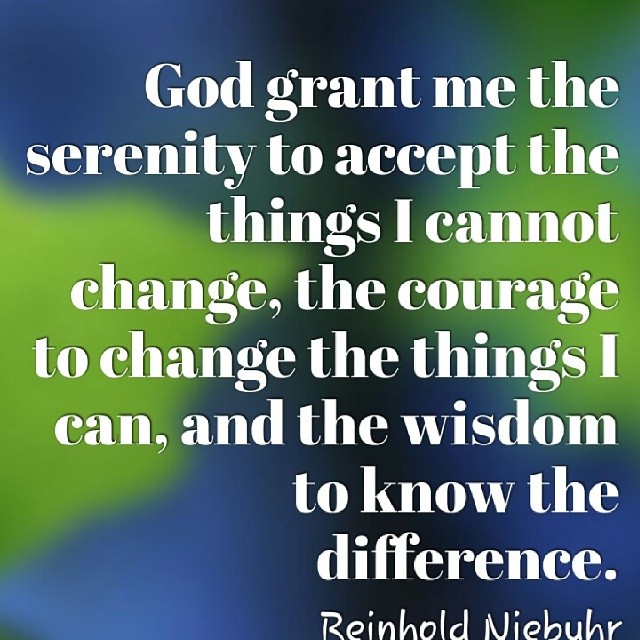This image features a computer-generated quote set against a blue and green gradient background. The background consists of wavy, splotchy patterns with a mix of lime green and ocean blue, blending together intricately, with darker blue tones centralized and lighter hues radiating outward. The quote, prominently displayed in large, white text, reads: "God grant me the serenity to accept the things I cannot change, the courage to change the things I can, and the wisdom to know the difference." At the bottom of the image, the quote is attributed to Reinhold Niebuhr, with his name appearing in smaller, white text in the lower right corner. The entire composition has a soft, somewhat blurry effect, likely crafted using Photoshop or other post-production software.